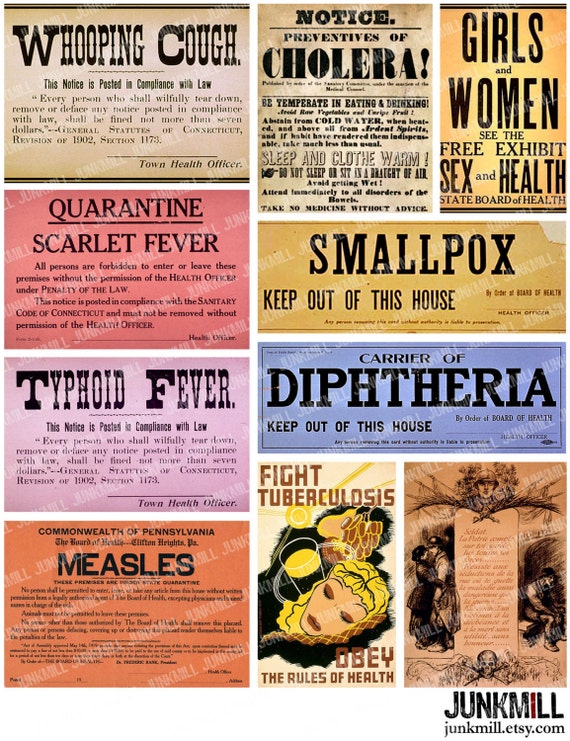This image is a collage of historical disease-related notices, compiled by JunkMill (junkmill.etsy.com). It features a variety of posters, each printed on different colored sheets of paper, including brown, red, yellow, and blue. The upper left corner prominently displays a notice about whooping cough, stating: "This notice is posted in compliance with the law. Every person who shall willfully tear down, remove, or deface any notice posted in compliance with this law shall be fined not more than $7." This is followed by legal references: "General Statutes of Connecticut, Revision of 1902, Section 1173, Town Health Officer." Adjacent to it is a preventative notice for cholera urging people to be temperate in eating and drinking, avoid cold water when heated, and refrain from taking medicine without advice.

To the right, another poster invites girls and women to a free exhibit on sex and health organized by the State Board of Health. Further below on the left, there are quarantine notices for scarlet fever and measles, both stressing legal penalties for entering or leaving the premises without health officer permission. Detailed warnings for typhoid fever and diphtheria assert similar legal consequences, emphasizing compliance with public health laws.

Notably, a bright red notice warns against entering a house affected by smallpox, and another poster advocates fighting tuberculosis by obeying health rules. A poster in the collage featuring a skull, soldier, and a woman hints at the broader societal impact of diseases, though the text is too small to read. The cohesive theme of the image reflects past public health efforts and legal enforcement against contagious diseases.